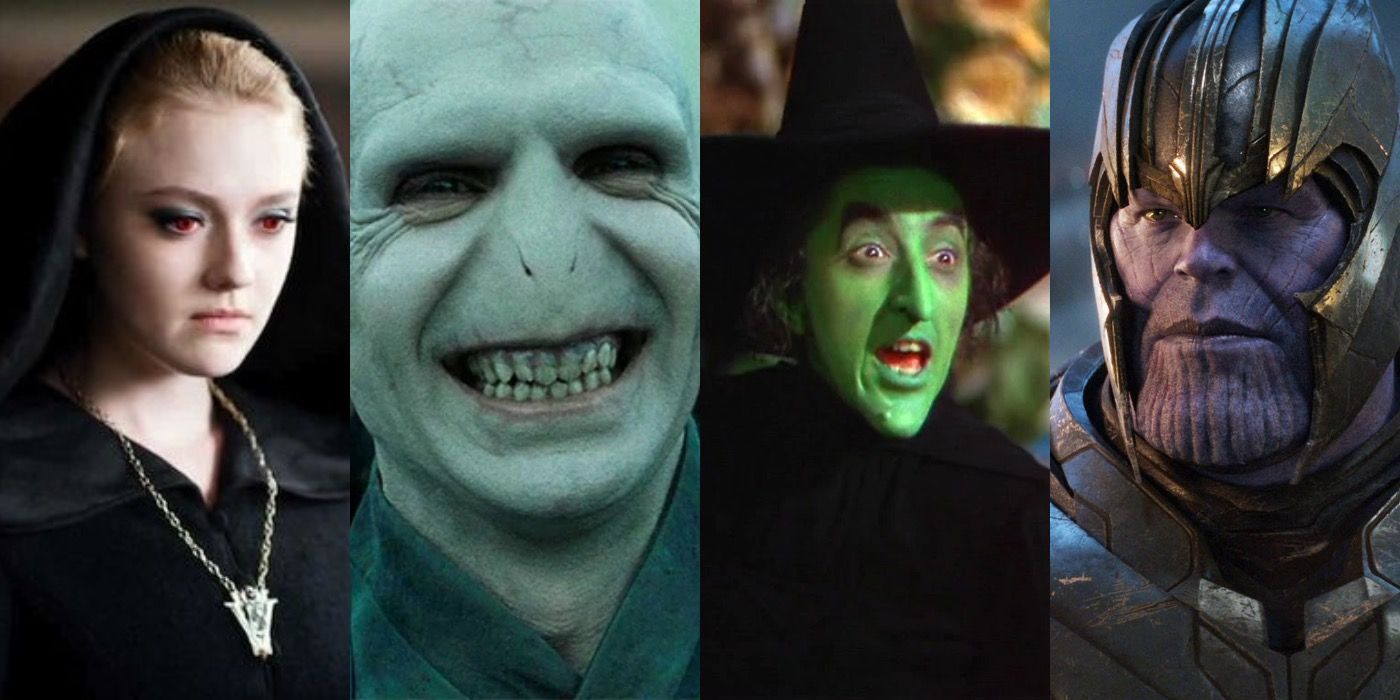The image is a collage featuring four characters from various movies, all of whom are iconic villains. On the left is a character who resembles a girl with short blonde hair, red eyes, and a serious expression. She wears a black cloak and a gold necklace and appears to be from the "Twilight" series. Next to her is Lord Voldemort from "Harry Potter," with his distinct snake-like appearance, gray washed-out skin, deeply wrinkled face, and grotesque smile revealing ugly teeth. The third character is the Wicked Witch of the West from the "Wizard of Oz," identifiable by her green skin, black witch hat, black outfit, and the signature mole on her chin; she is depicted with a surprised look. The fourth character is Thanos from the "Avengers" series, featuring his purple skin, defined facial structure with lines, and battle-worn scarring. He is dressed in armor and a metallic helmet.